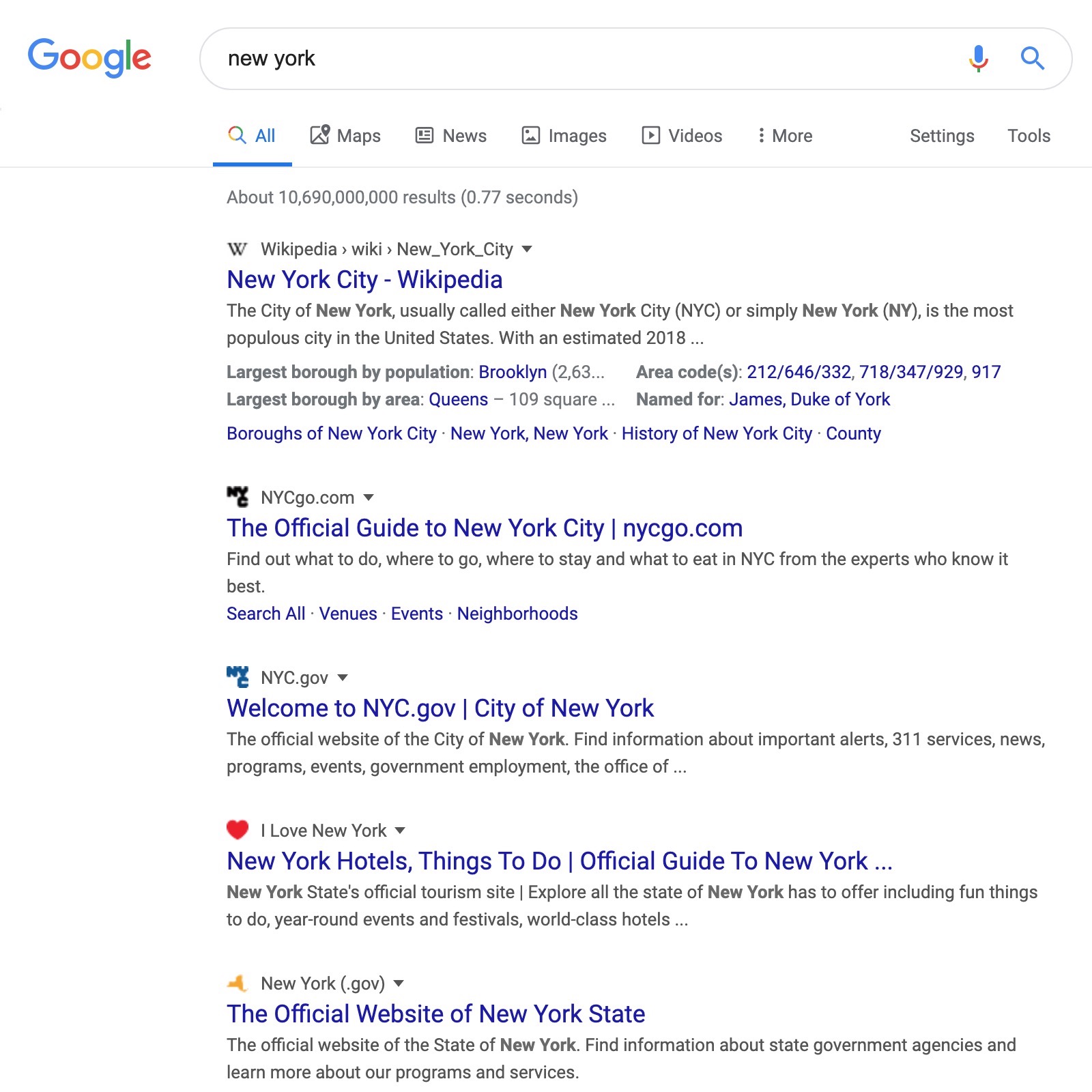This image captures a Google search results page with the classic Google logo prominently displayed in the top-left corner. In the search bar, the user has entered the query "New York." Below, Google reports a staggering 10,000,690,000,000 results found in approximately 0.77 seconds. 

The top result is a link to the Dutch version of Wikipedia, featuring the title "New York City - Wikipedia." This entry explains that New York City, also known by its initials NYC or simply as New York, is the most populous city in the United States with an estimated population in 2018. However, the text is cut off mid-sentence. Additional details briefly mention that Brooklyn is the largest borough by population and Queens by area.

Following this, the second result is the official website of the city of New York, listed as "Welcome to NYC.gov - City of New York." This site serves as the main portal for official information and services provided by the city government.